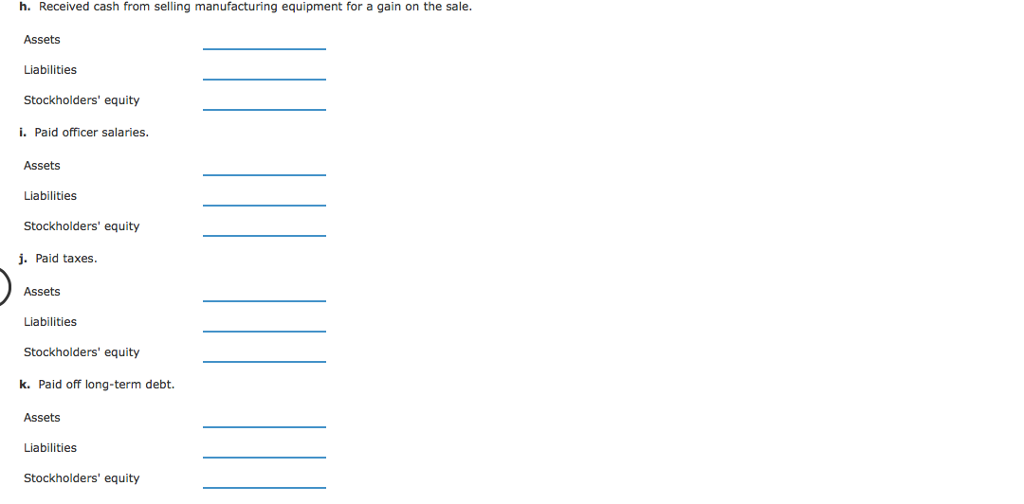The image appears to be a screen capture from a digital device, displaying a list of financial transactions and their associated accounting categories. At the top, item "h." is labeled "Received cash from selling manufacturing equipment for a gain on the sale." Beneath this header, three options are listed: 
1. **Assets** (marked by a blue line to the right)
2. **Liabilities** (marked by a blue line to the right)
3. **Stockholders' Equity** (marked by a blue line to the right)

Next, item "i." reads "Paid officer salaries." Similarly, underneath this, three options are available:
1. **Assets** (marked by a blue line to the right)
2. **Liabilities** (marked by a blue line to the right)
3. **Stockholders' Equity** (marked by a blue line to the right)

Subsequently, item "j." is titled "Paid taxes," with the same three options listed beneath it:
1. **Assets** (marked by a blue line to the right)
2. **Liabilities** (marked by a blue line to the right)
3. **Stockholders' Equity** (marked by a blue line to the right)

The final listed item, "k.," states "Paid off long-term debt." As with the previous items, the three accounting categories are presented:
1. **Assets** (marked by a blue line to the right)
2. **Liabilities** (marked by a blue line to the right)
3. **Stockholders' Equity** (marked by a blue line to the right)

The blue lines to the right of each option suggest a selection mechanism, possibly indicating that these options can be chosen or interacted with for categorization purposes.